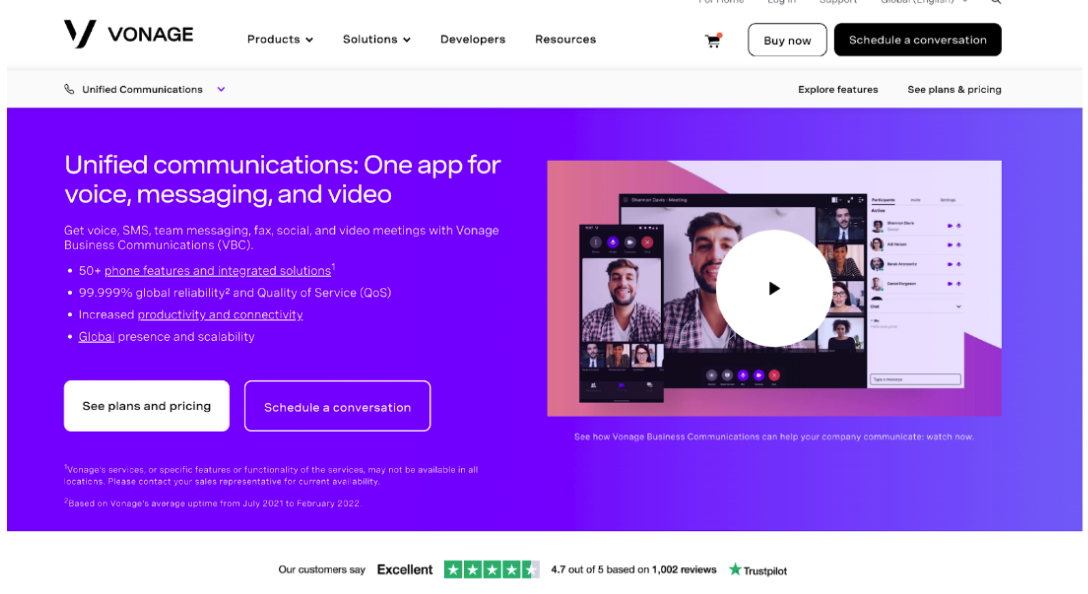The image features the Vantage website interface. In the upper left corner, the brand name "Vantage" is displayed. Navigation options stretch across the top, including "Products" with a drop-down menu, "Solutions" with another drop-down, "Developers," "Resources," and a shopping cart icon on the far right adorned with a red circle. To the right of the navigation, there's a white "Buy Now" button outlined in black with black text, and a black "Schedule Conversation" button with white text.

Below the navigation bar is a gray line. On the left side, it reads "Unified Communications" with a drop-down menu. On the right, options include "Explore Features" and "See Plans and Pricing." 

Beneath this section lies a purple horizontal rectangle. On the left side, in white text, it states: "Unified Communications: One app for voice, messaging, and video." It also lists the following features: "Get voice, SMS, team messaging, fax, social, and video meetings with Vantage Business Communications (VBC)." Bullet points highlight key benefits: 
- "50+ phone features and integrated solutions"
- "99.99% global reliability and quality of service (QoS)"
- "Increased productivity and connectivity" 
- "Global presence and scalability," with the words "productivity," "connectivity," and "global" underlined for emphasis.